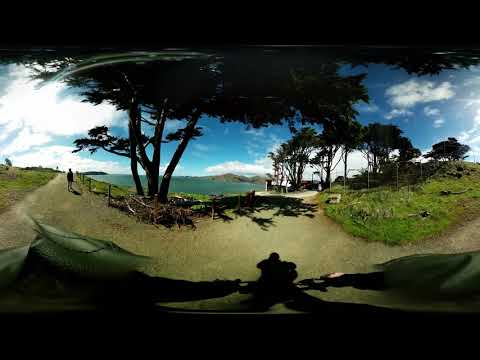This outdoor photograph captures a picturesque scene of a tropical or park-like setting, likely an island or coastal area. The central feature is a tan, sandy walking path that starts from the foreground, curves gracefully to the left, and eventually bends back towards the center-right of the image. A person, possibly riding a bike, is visible in the distance on this path. In the mid-ground, a solitary tree stands to the right of the path, while a cluster of trees with tall, thin trunks and heavy canopies is visible further to the right, on a gentle incline. 

The left side of the image predominantly shows more of the walking path and the person traveling along it. In the distant background, a body of water, possibly a lagoon, bay, or the ocean, extends to meet the horizon. The water appears dark blue, contrasting with the lightly clouded, light blue sky above, which takes up the top half of the image. The scene is bathed in bright sunlight, casting long shadows of the trees and the person, emphasizing the natural beauty and tranquility of this almost deserted location. The overall setting feels like a serene retreat, perfect for leisurely walks or rides along the scenic path near a peaceful waterway.